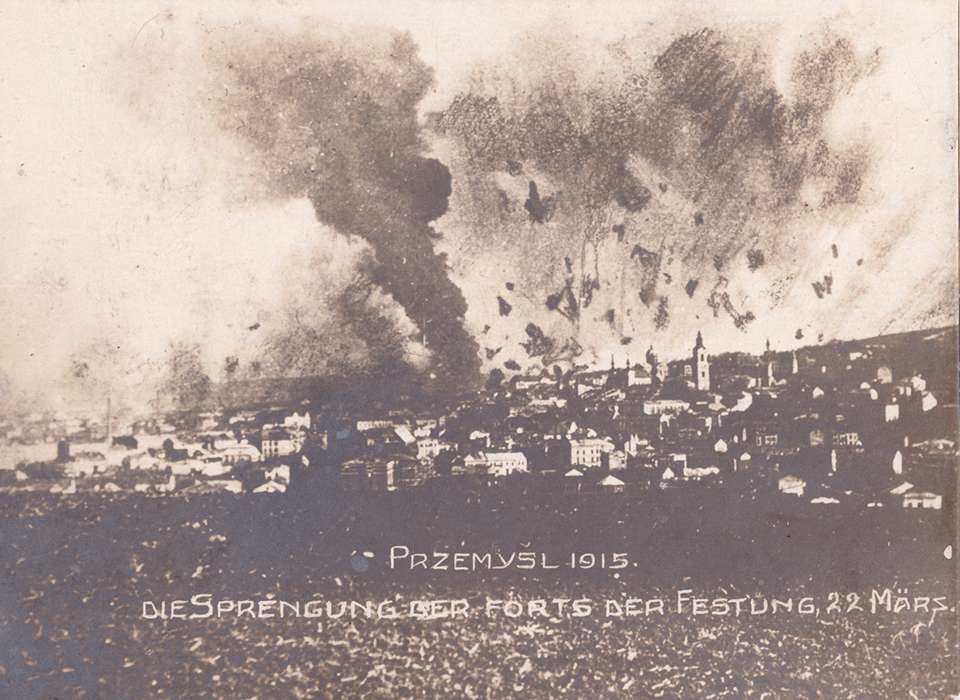This black and white photograph captures a dramatic and devastating scene of the city of Przemysl under attack on 22 March 1915. The image is partly faded and yellowed with time, underscoring its historical significance. The city’s European-style buildings, all in white, stand in stark contrast to the very dark and blurry foreground, which appears to be a field. Visible in the center and background of the photograph, the city is enveloped in chaos, with thick black smoke billowing from multiple points and particularly heavy plumes rising from a massive explosion. Debris, large and clearly from a severe bombing presumably linked to World War One, can be seen scattered in the air. The text at the bottom reads "PRZEMV5L 1915" and "DAISPRENGUNDERFORTSDERFESTUNG 22 MARS," indicating this photograph records "Die Sprengung der 4. der Bestung," marking the date of the fort's explosion. This image vividly portrays the catastrophic impact of warfare on the city of Przemysl, evidencing a significant event during World War One.